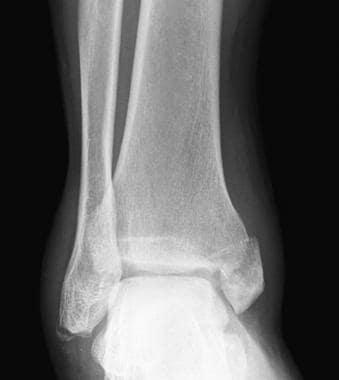This detailed portrait-oriented x-ray image reveals the intricate structure of a human leg. The image captures a knee joint, where the femur, tibia, and fibula are clearly visible. The femur rises from the bottom and connects to the knee joint, where it meets the tibia and fibula, both extending upward. The bones are depicted in shades of light gray to white, typical of x-ray imaging, surrounded by faint, smoky-like tissue representations against a stark black background. This x-ray prominently showcases the anatomical alignment and connection of the major leg bones within the knee joint.